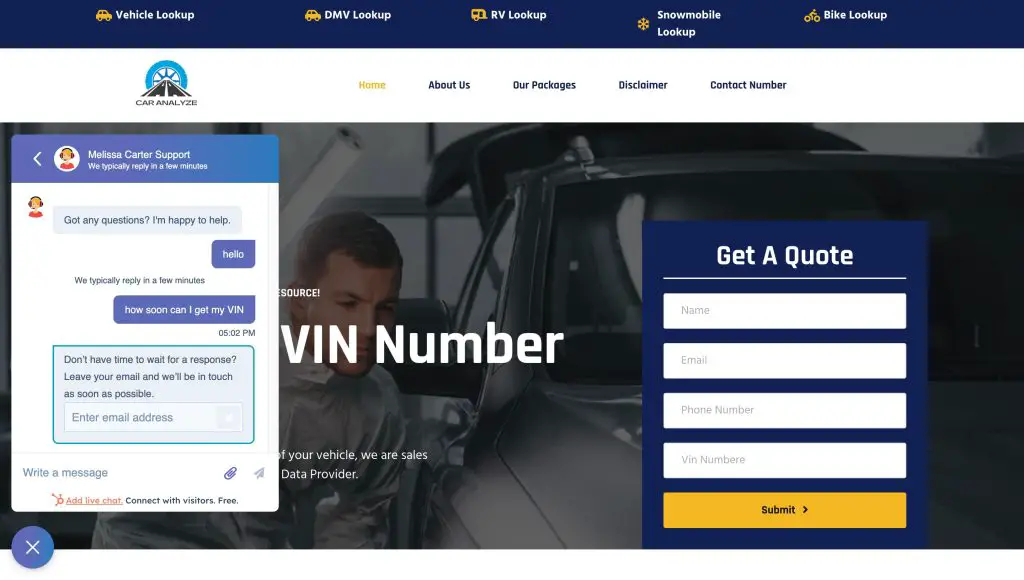The screenshot from the Car Analyze website displays a navy blue header at the top, which features clickable options from left to right: "Vehicle Lookup," "DMV Lookup," "RV Lookup," "Snowmobile Lookup," and "Bike Lookup." Beneath this, the Car Analyze logo is prominently showcased, depicting a road stretching into the distance with the sun rising over the horizon. This logo area has a white background. Below the logo, there are navigation tabs in orange and black text, including "Home" (in orange), "About Us" (in black), "Our Packages" (in black), "Disclaimer" (in black), and "Contact Number" (in black). 

Taking up the lower portion of the screen is a large image of a man kneeling to inspect a gray-colored car. To the right of this image is a navy blue square box labeled "Get a Quote," which contains fields for users to input their information.